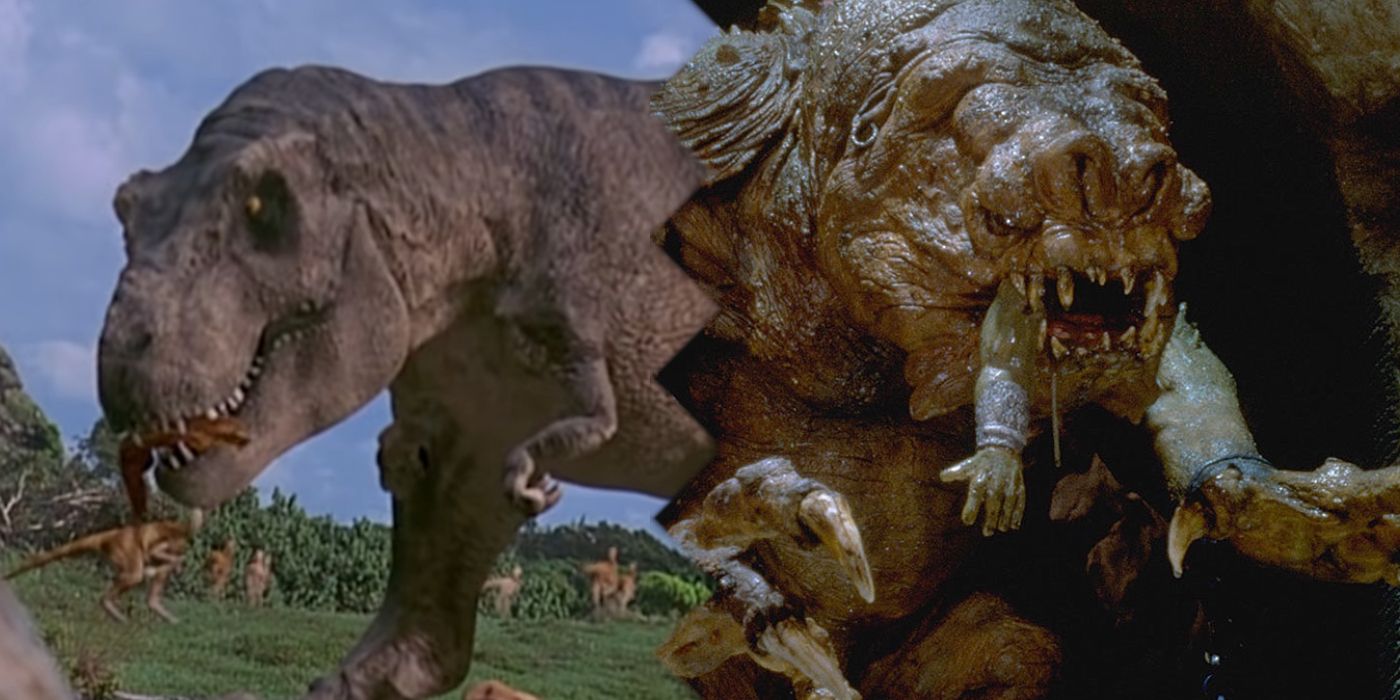In this vivid image, the left side features a prominent grayish-brown dinosaur with a massive head, its mouth holding a much smaller dinosaur. It has notably short and tiny front limbs and is oriented facing left. This scene is set against a rich blue sky with green grass covering the field, where additional smaller dinosaurs, resembling kangaroos in form and bright brown in color, can be seen frolicking and some even jumping in the background. Trees dot the landscape, enhancing the prehistoric atmosphere. On the right side, the focus shifts to an imposing brown dragon with a shiny exterior. It looks enraged, its mouth wide open to reveal a set of irregular, long teeth. The dragon has two front arms—one resembling a human hand and the other resembling a larger animal limb—with the left arm extending near its mouth, adding to its fierce appearance.